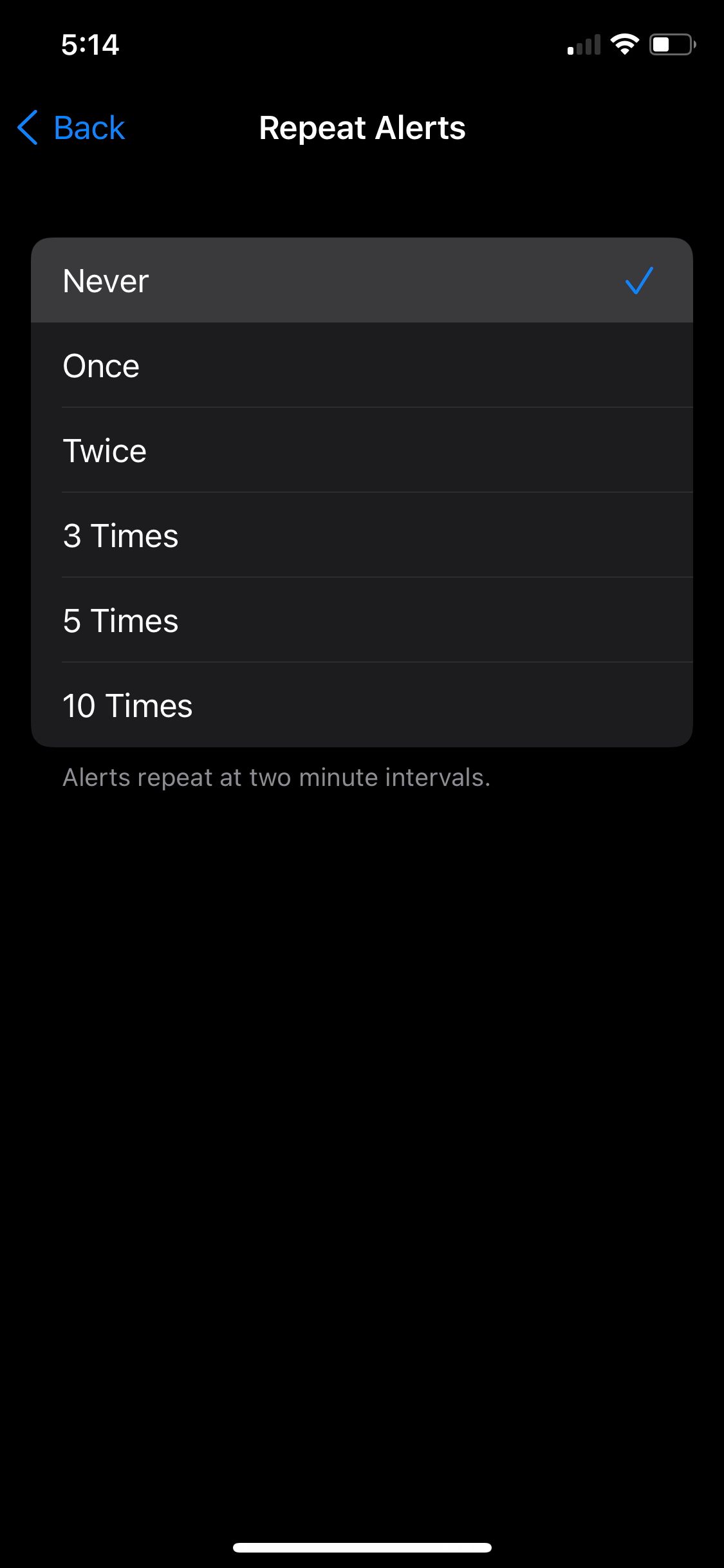In the image, set against a black background, a prominently displayed blue number "514" accompanied by a left-pointing arrow stands out. Positioned above, "Repeat Alerts" is distinctly written in white text. Below this heading, a chart is featured with various options for setting alert intervals. The option "Never" is highlighted in a light gray rectangle, contrasting the dark gray rectangles that frame the remaining choices. To the right of this gray section, a blue check mark indicates a selection. The chart lists several alert intervals: "Once," "Twice," "Three Times," "Five Times," and "Ten Times," each specifying notifications to repeat at two-minute intervals. At the bottom-left corner of the image, there is a bar that appears more white than gray, adding to the structured layout of the graphical elements.